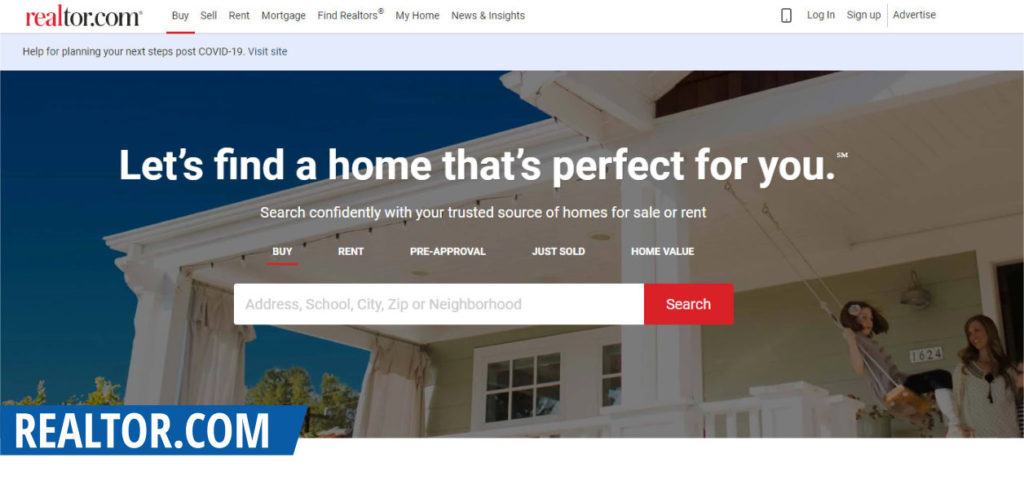The top left corner features the logo "Realtor.com" with "R-E-A-L" in red and the remaining letters in black. Adjacent to the logo are navigational options including "Buy" (underlined in red), "Sell," "Rent," "Mortgage," "Find Realtors," "My Home," "News & Insights." Approximately five inches to the right, there is an icon of a cell phone followed by "Log In," "Sign Up," a small vertical line, and "Advertise." Below this section, a long blue line displays the text: "Inside help for planning your next steps post COVID-19" with a blue clickable option labeled "Visit Site."

The main image depicts a white front porch with a girl swinging on it and a woman standing to her right. The left side of the image has a blue sky background. Overlaid text reads: "Let's find a home that's perfect for you. Search confidently with your trusted source for homes for sale or rent." Below this, options include "Buy" (underlined in red), "Rent," "Preapproval," "Just Sold," and "Home Value." Beneath these options is a white search bar with a red "Search" button next to it. The far left corner features the "Realtor.com" logo in all capital letters within a blue box.